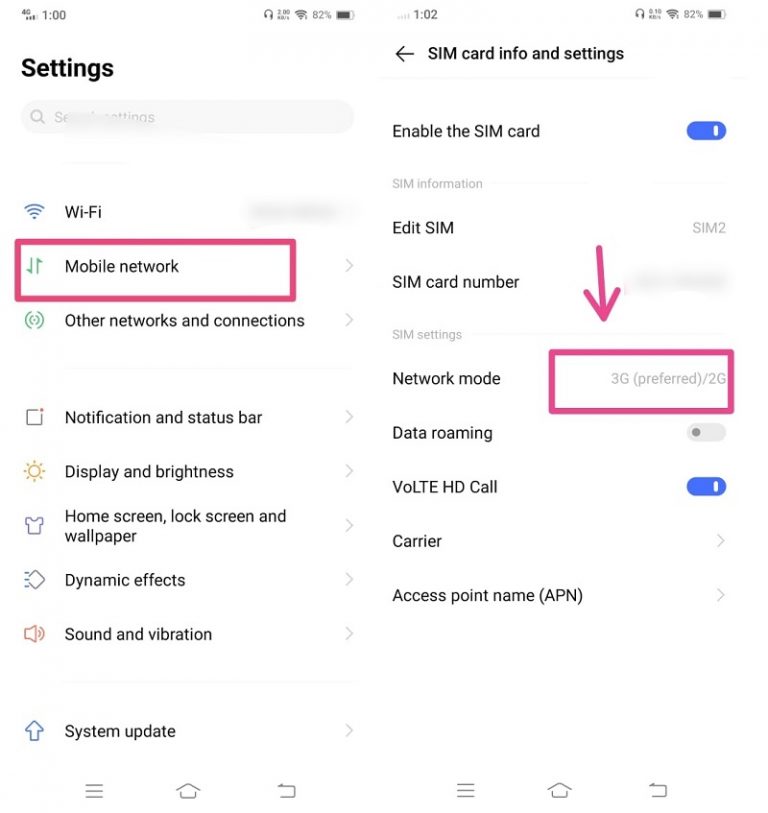The image consists of two side-by-side screenshots from an Android mobile device, showcasing a step-by-step navigation through the settings menu. 

The first screenshot displays the general settings page within the Android Settings app. The entries visible include “Wi-Fi” at the top, followed by “Mobile network.” A pink box has been digitally added around “Mobile network,” indicating it as the selection point. 

The second screenshot appears sequentially, illustrating what is shown after “Mobile network” is selected. This page is titled “SIM card info and settings,” with a back arrow at the top. The settings include options like “Enable the SIM card” (toggled on) and “Edit SIM.” A pink arrow points downward to a highlighted section within a pink box, which is labeled “Network mode.” The highlighted setting within this box is “3G preferred/2G.” 

Both screenshots feature a clean, white background, making the text and highlightings easy to read.